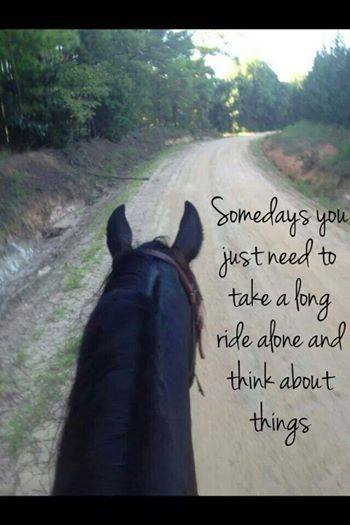The photo presents a first-person perspective from atop a horse with a prominent view of its black head and mane. The scene depicts a light gray to light brown dirt road flanked by gentle, sloping hills that give way to dense tree lines on both sides. The horse, which has black fur, appears to be navigating this slightly elevated path, revealing a serene, shaded trail bordered by green grass and vegetation. Black cursive text to the right of the image poignantly reads, "Some days you just need to take a long ride alone and think about things."